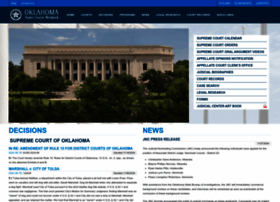The image is a low-quality screenshot of a web page, with a very small size and hard-to-read fonts. The layout, however, can still be discerned. At the very top, a narrow blue border is followed by a slightly wider, darker blue border. In the upper left corner, the text appears to say "Oklahoma," with some unreadable text beneath it. Next to this, there is a gray circle, with the "Oklahoma" text also in gray, and the center of the circle contains a gray star shape.

The menu items are listed in a gray font, but due to the blurry and small size, they are unreadable. Below these headers, the top half of the page is dominated by a large photo of a building with a light gray surface, resembling a federal or municipal structure. On the right side of the page, there's another menu within a white box with blue font that is unfortunately not readable.

Under the photo on the left side, bold blue text spells out "Decisions," followed by "Supreme Court of Oklahoma" in a darker blue font, but further text is not legible. On the right side of the page is a column with the headline "News" in blue, but the content beneath this header is also unreadable.